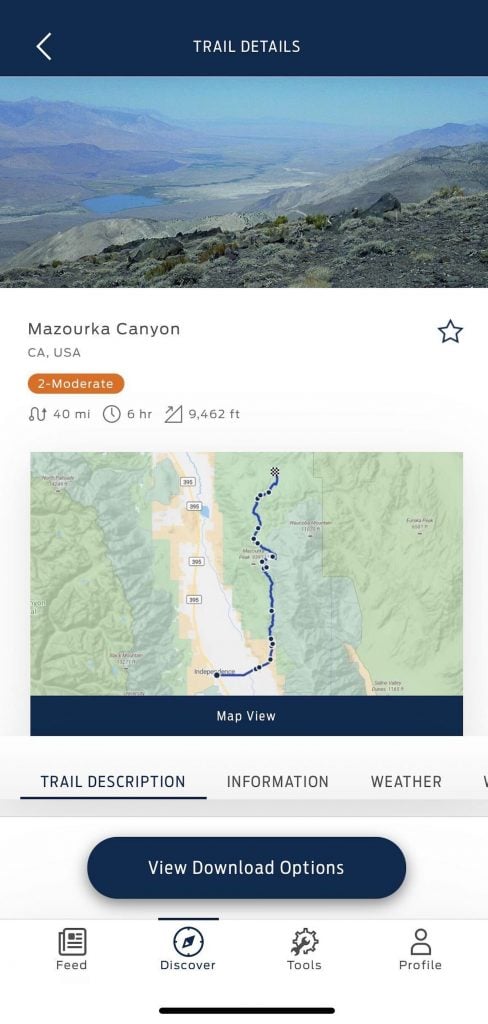This is a detailed description of a website screenshot, captured on a smartphone in portrait orientation. At the top of the screen, the webpage title "Trail Details" is displayed in white text. On the top left corner, there is a back arrow icon, allowing users to navigate back to the previous page.

The upper portion of the screenshot features a landscape image. On the top left of the image, there's a sunlit desert-like region with a small lake in the middle. In contrast, the bottom right part of the image showcases a landscape predominantly covered in trees, with possible houses or trails scattered among the grassy area, which is less sunlit.

Directly below the landscape image, the text "Mazorca Canyons" is displayed, indicating the name of the location, followed by "California, USA" to specify its location. Beneath this information, "Moderate" is highlighted on an orange background, signifying the difficulty level of the trail. Further down, details about the trail are provided: "40 mi", "6 hours", and "9,482 feet", suggesting that the trail is 40 miles long, takes approximately 6 hours to complete, and has an elevation of 9,482 feet.